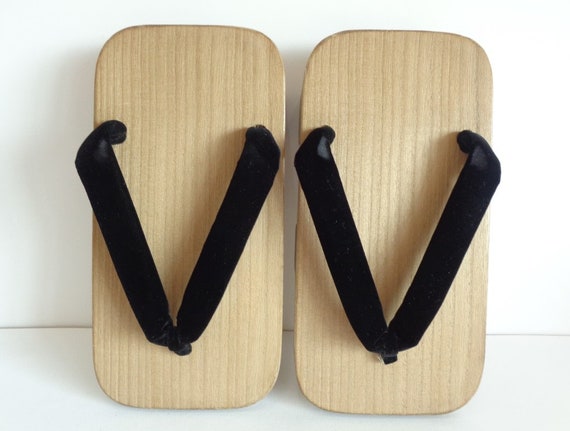Here is an image depicting what appears to be a pair of wooden flip-flops. The flip-flops are light tan in color, constructed from a pale wood with lines that are a slightly darker tan. They feature thick black straps that form a V shape, attaching from either side to the center towards the toes. The flip-flops are rectangular in shape, having equal width from front to back, and they do not taper. The background consists of a white wall and a very light gray surface, likely a table, on which the flip-flops are leaning. Small shadows are cast to the left, adding depth to the scene. These flip-flops resemble traditional wooden clogs but with a modern twist, possibly suggesting a novel take on footwear, perhaps inspired by designs seen in tourist spots like Amsterdam.